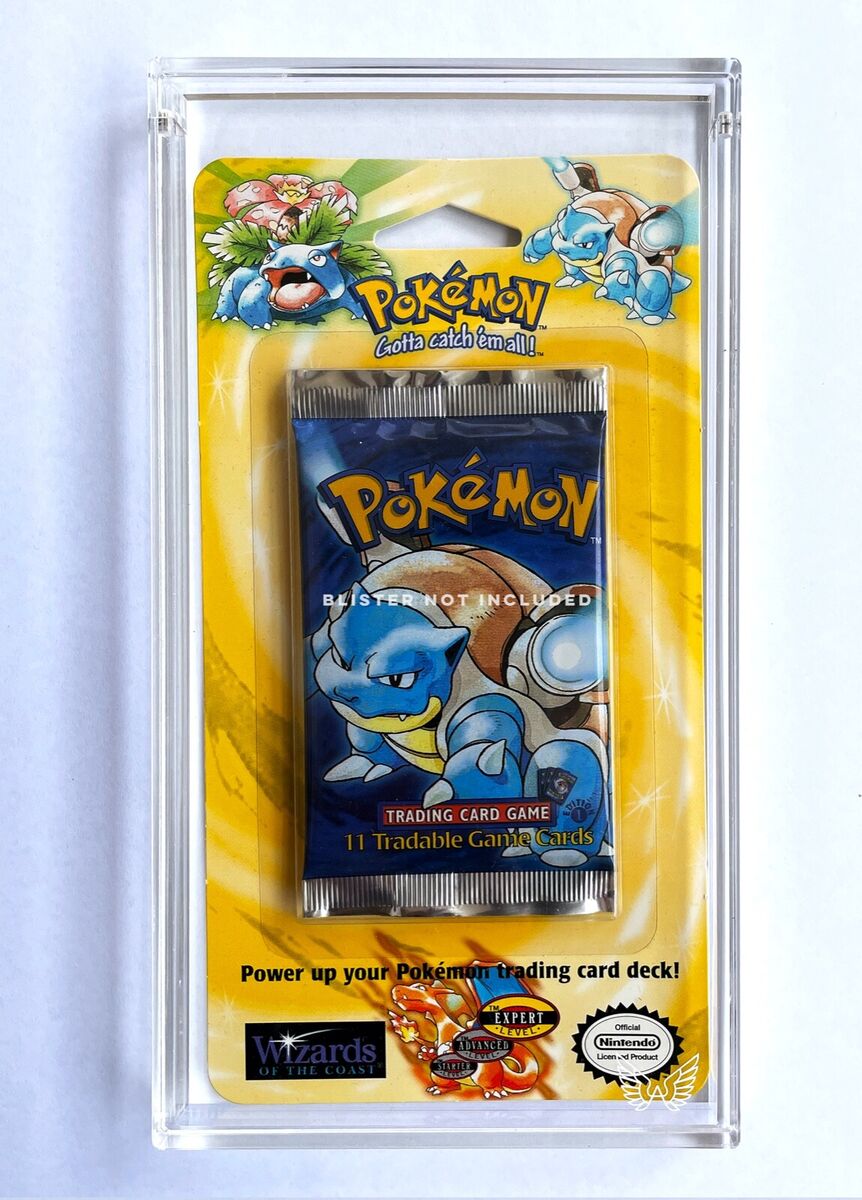The image showcases an unopened pack of Pokemon trading cards encased in a clear plastic case, mounted on a yellow backboard. The foil package inside prominently features the name "Pokemon" along the top, and a turtle-like Pokemon with a blue face and ears on its cover. Across the package, white text reads "Blister not included," and below that, it says "Trading Card Game, 11 tradeable game cards." The yellow backboard mirrors the package design, displaying the same turtle-like Pokemon on the upper right and an additional variant with a plant on its back on the left. At the bottom of the card, against an orange dragon backdrop with ovals, it says "Power Up Your Pokemon Trading Card Deck," followed by labels indicating "Expert Level, Advanced Level, Starter Level." Company logos, including "Wizards of the Coast" and "Official Nintendo Licensed Product," are also present near the bottom. The entire setup stands out against a light bluish background with a small flowery design to the right.